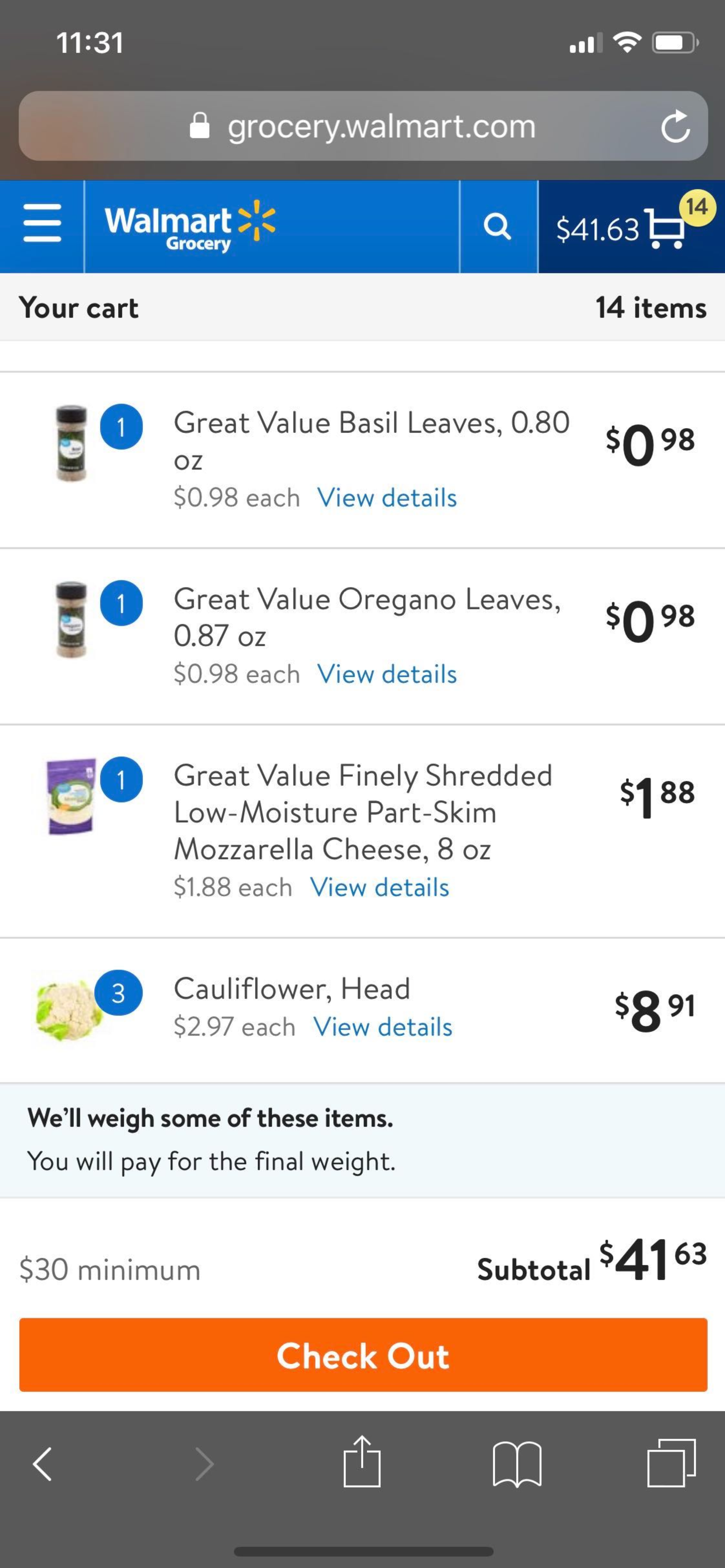This image is a screenshot from a cell phone displaying a Walmart Grocery cart. 

At the top, the banner is a charcoal gray background featuring white text. In the left-hand corner, it shows the time as 11:31, while the right-hand corner displays icons for cell signal, Wi-Fi signal, and battery level.

Below this banner, there's a search bar with a padlock icon and the URL "grocery.walmart.com." To the right, a refresh icon is visible. 

The following section consists of a light blue banner with three horizontal white lines stacked one over the other, accompanied by the text "Walmart Grocery." Next to this is a magnifying glass icon representing a search function. Beside it, a dark blue rectangle displays "$41.63" next to a shopping cart icon. A small yellow circle with the number "14" in it is affixed to the cart icon, indicating the number of items in the cart.

The background then transitions to light gray, displaying the heading "Your Cart, 14 items." Below this heading, a list of some of the items in the cart includes "Great Value Basil Leaves," "Great Value Oregano Leaves," "Great Value Finely Shredded Low Moisture Part-Skim Mozzarella Cheese," and "Cauliflower Head."

Additionally, a note indicates that some items' weights will be calculated, with a "$30 minimum" requirement specified. The subtotal for the cart is mentioned as "$41.63."

At the bottom, a prominent orange banner captioned "Checkout" is present, guiding users to proceed with their purchase.